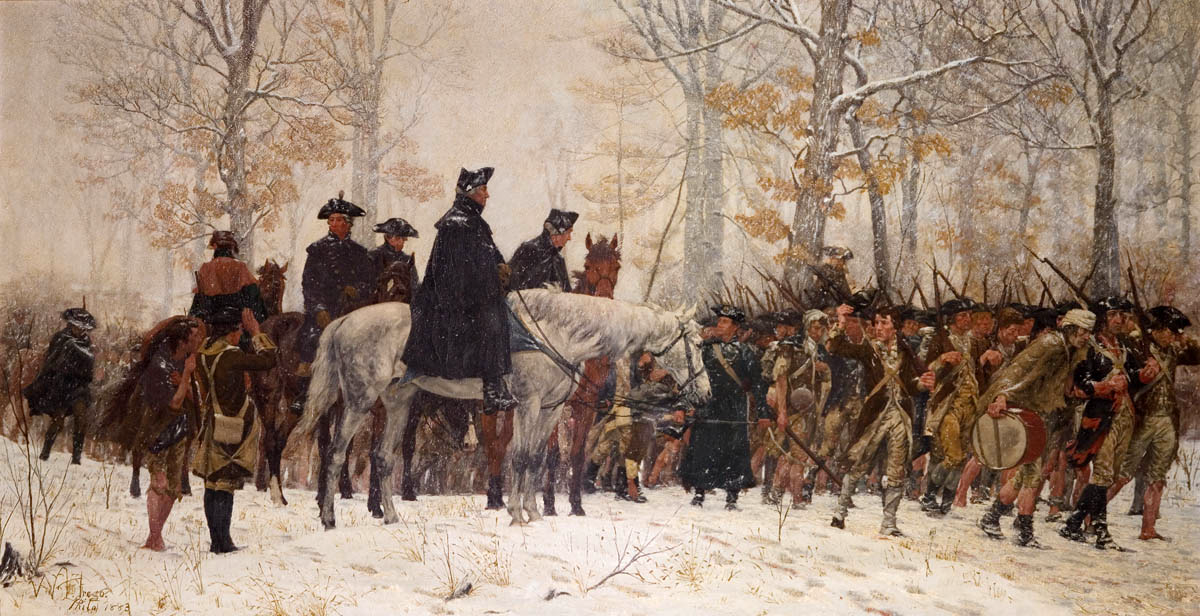This painting, likely from the Revolutionary War period in the late 1700s, depicts a winter battle scene. The setting is outdoors with snow covering the ground, through which yellowed and brown grasses poke. The sky is snowy, and the trees in the background have lost most of their leaves, with the remaining foliage a mix of orange and brown, set against visible brown trunks. The men, clad in military uniforms, are preparing for combat. Some soldiers are equipped with rifles and bayonets, while others carry drums. Central to the scene is a commanding figure, possibly George Washington, mounted on a white horse, dressed in a black coat and hat. Nearby, another soldier is saluting, adding to the sense of military preparation and determination evident in the scene.